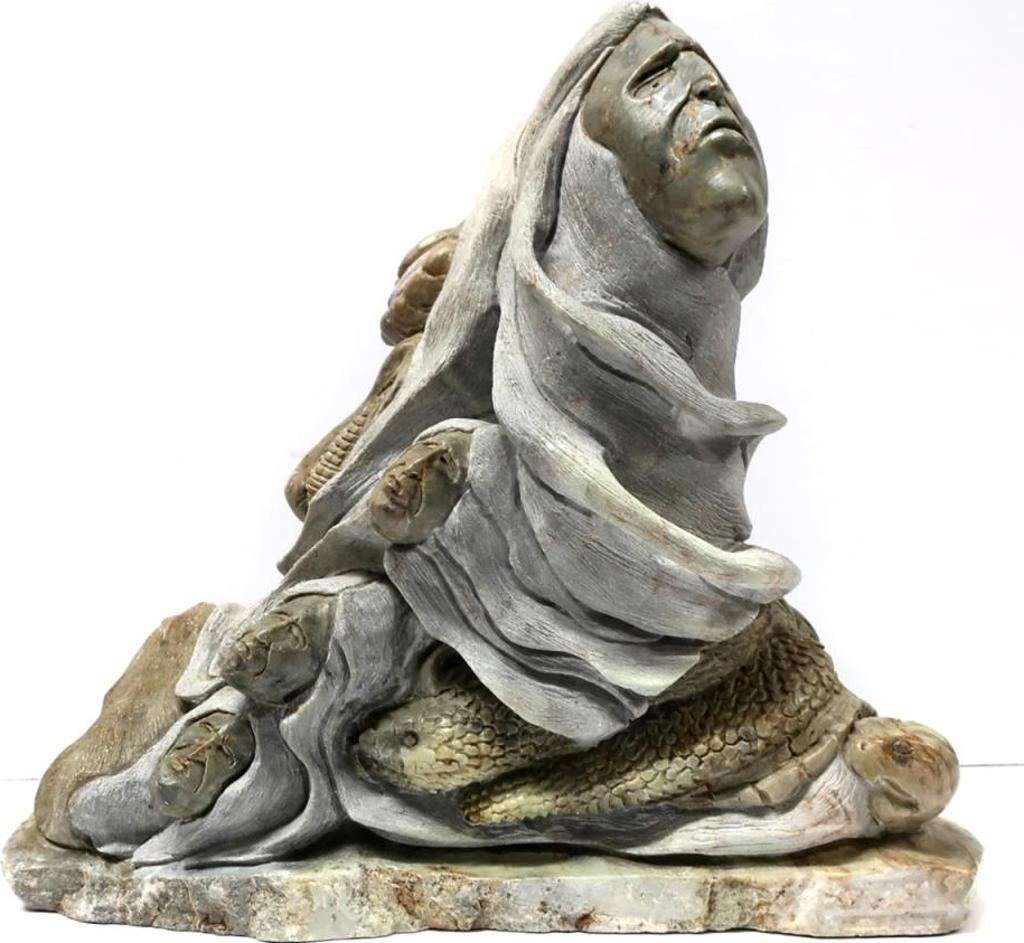The photograph captures a highly abstract, triangular-shaped sculpture crafted from a combination of white, marble-like stone with hints of brown and silver. The statue features a prominent, large human face at the apex, gazing upwards and to the right, draped in a billowing scarf or linen cloth that cascades down and intertwines with the rest of the sculpture. Below this main face, there are three smaller faces oriented to the left. These faces seem to emerge from within the sculpture, blending seamlessly into the surrounding material, emphasizing the piece's abstract nature. Further down, coiled at the base and partially visible, is a detailed depiction of a snake, characterized by its scaly texture and a visible eye. The base of the sculpture, which secures it, blends with the overall light marble hue of the piece, enhancing its ethereal and uncommon aesthetic. All elements combined contribute to the statue's majestic and enigmatic presence.